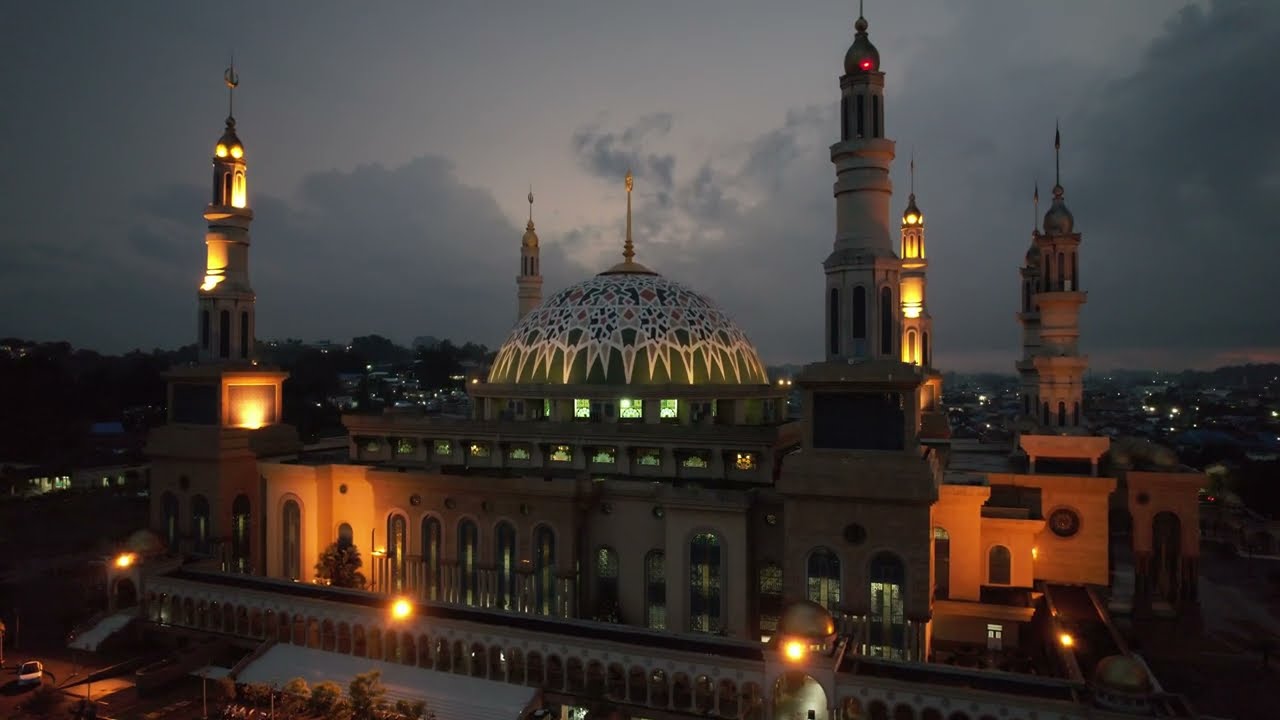In this nighttime image, an imposing and intricately designed building, possibly a significant landmark, dominates the center. The structure resembles a large synagogue or an oriental palace with a central dome featuring a checkered pattern of green and beige, capped by a pointy spire. Flanking the dome are multiple tall, needle-like towers—counting seven in total, each with pointed tops. The wide building is adorned with numerous tall, rounded windows and is enclosed by a concrete fence with lights illuminating its lower sections. The background reveals a dark, cloudy sky, blending gray shades with black shadows cast by distant buildings and trees, suggesting a late evening setting. The color palette includes yellow lights, green, tan, red, white, black, and gray hues, creating an atmospheric and dramatic nighttime scene.